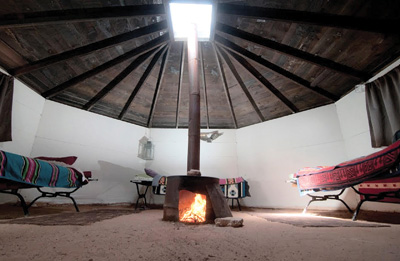The image depicts the interior of a cozy, makeshift cabin with an octagonal or pentagon shape, reminiscent of a giant teepee or tent. The white-plastered walls are contrasted by a dark wooden ceiling that converges at the center, where a metal pipe from a wood stove extends through an opening at the top. The floor appears to be made of dirt, contributing to the rustic atmosphere. Inside, there are three rudimentary single mattress cots: one with a red mattress, another with a blue mattress and a purple blanket, and a third one further ahead. A sense of warmth and simplicity permeates the space, enhanced by the central wood stove that promises to make this unconventional dwelling a cozy retreat. The presence of windows with curtains and the description of a sunlight effect emphasizes the blend of natural lighting and practicality in the design.